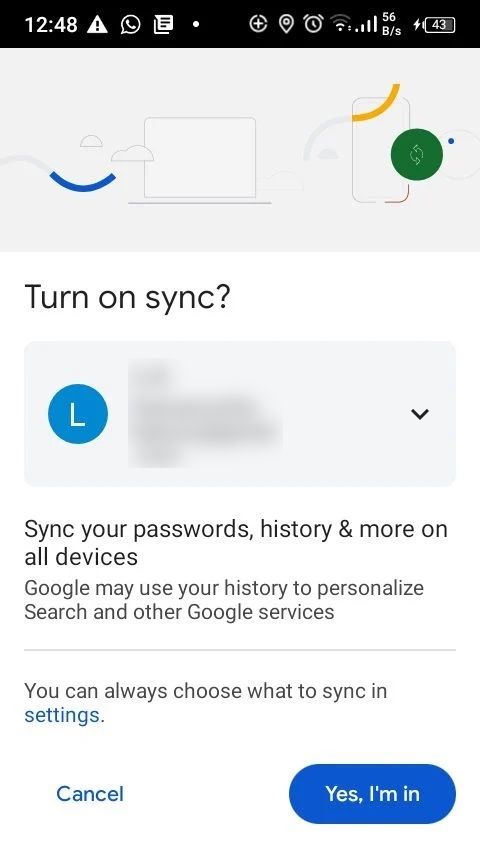This image is a screenshot from a smartphone showing a notification screen. The top header is black with white font: the time is displayed in the upper left corner as 12:48, and the battery icon in the upper right corner shows a 43% charge. Additional icons include a phone, messaging, an active alarm, and Wi-Fi, which has a low signal strength indicated by only two bars being lit.

Directly below this header is a light gray graphic banner featuring a simple line drawing of a computer screen and a smartphone. A green filled circle is also present. Beneath this, against a white background, the text "Turn on sync?" appears in gray font.

Further down is a very light blue-gray rectangle containing a blue circle with a white "L" in the middle. This area seems to have had the user's name and other account details blotted out with gray for privacy. Below this, in gray font, it says, "Sync your passwords, history, and more on all devices," followed by a brief explanation.

At the very bottom right corner, there is a blue button with rounded corners that says, "Yes, I'm in" in white text.